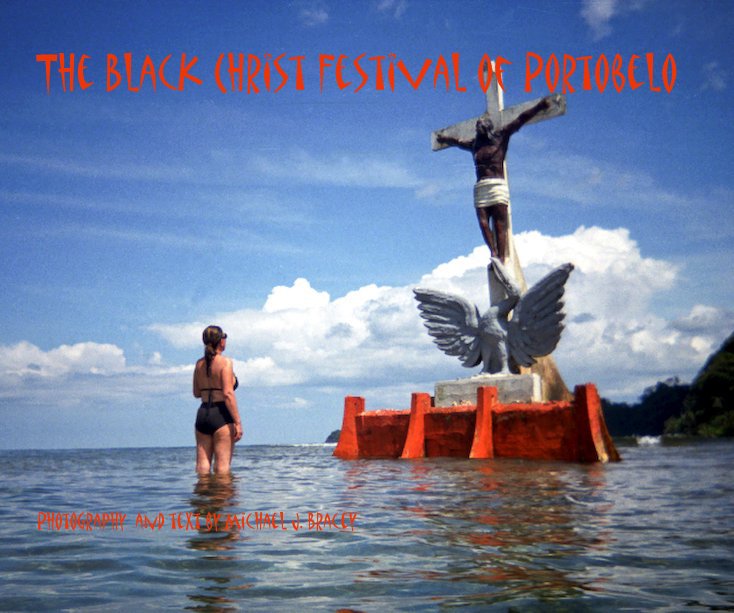In this photograph taken with an auto setting, the scene captures a serene body of blue water, possibly an ocean, with remarkably calm surface conditions. Dominating the center of the image is a striking statue of a black figure of Christ on a white wooden cross. At the base of the crucifix stands another statue, this one of a green bird with its wings spread wide, possibly resembling a stork or pelican. The statues are mounted on an orange platform that appears to be partially submerged in the water.

To the left of the statues, a woman stands knee-deep in the water. She is dressed in black swimwear and her hair is tied back in a ponytail. She gazes intently at the statues, her legs submerged up to the knees while the rest of her body remains above the waterline.

The sky above is a clear blue with scattered white clouds, adding to the tranquil atmosphere of the scene. Overlaying the top of the image is red text that reads, "The Black Christ Festival of Portobello," while in the bottom left corner, in smaller text, it states, "Photography and text by Michael J. Bracey."